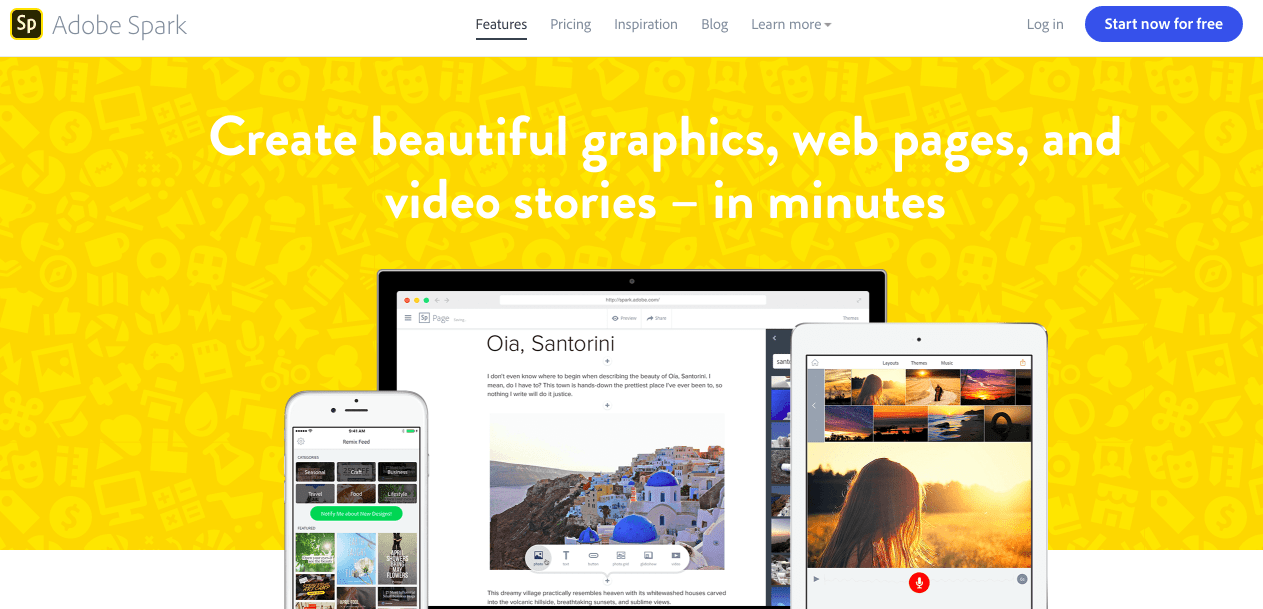The screenshot features a website for Adobe Spark. Central to the image is a black square emblazoned with the yellow letters "S" and "P". Above, a navigation menu displays options for "Features", "Pricing", "Inspiration", "Blog", and "Learn More," with "Features" currently underlined, indicating it is selected. To the right of the navigation bar, there are buttons labeled "Log In" and "Start Now for Free," with the latter highlighted in yellow.

The main section of the screen is dominated by an eye-catching banner. A yellow rectangle contains several images and, written in elegant white font, the text reads: "Create beautiful graphics, web pages, and video stories in minutes."

Below the banner, the webpage showcases images of the Adobe Spark application interface displayed across various devices, including a smartphone, an iPad or tablet, and a desktop computer. On the desktop interface, the text "Oi Santorini" (spelled "O-I-A, S-A-N-T-O-R-I-N-I") is visible, accompanied by an image likely depicting the picturesque city of Santorini.